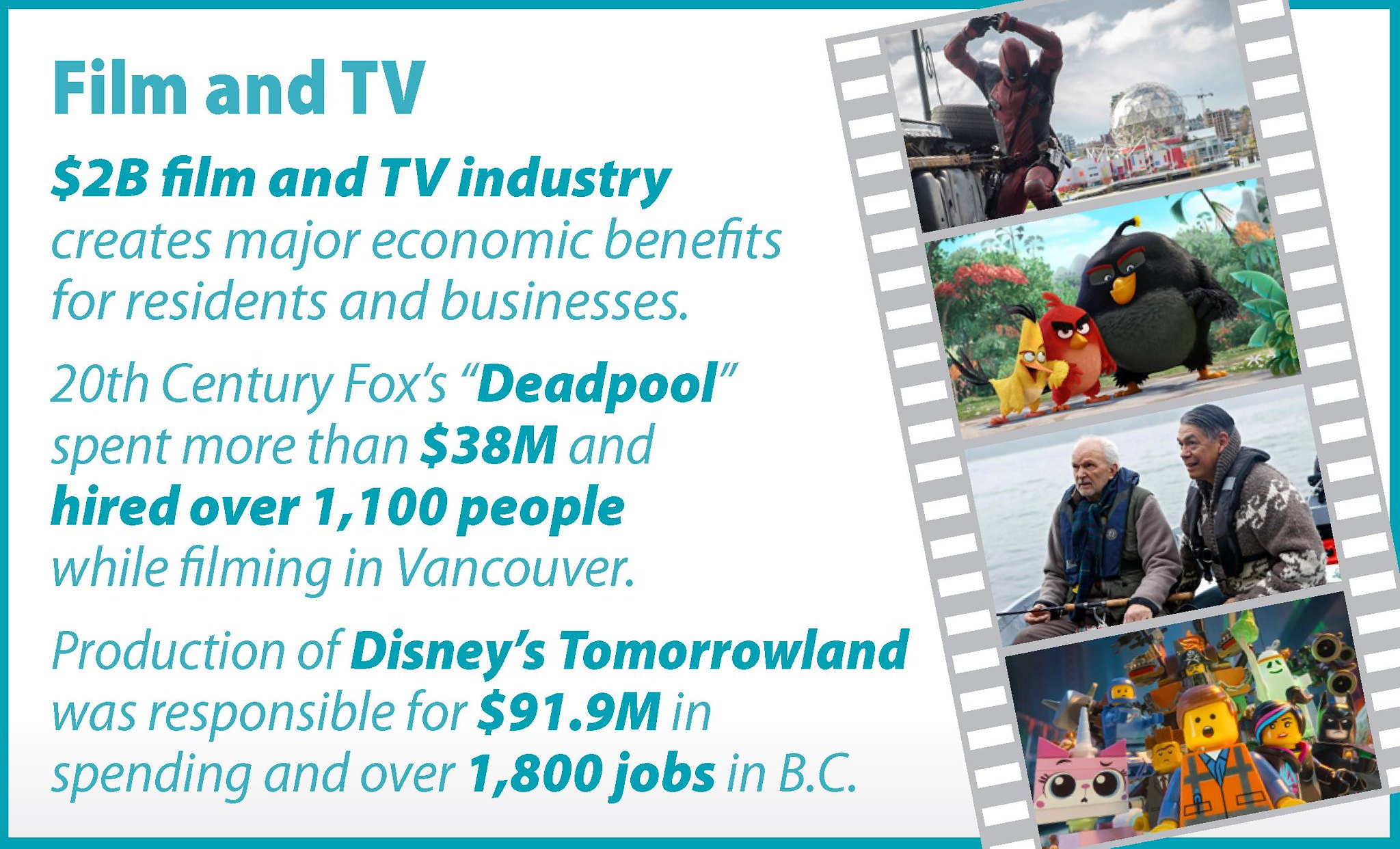The image is a horizontally oriented rectangular advertisement with a white background and a blue border. On the left side, it features detailed blue text that highlights the significant economic impact of the film and TV industry, valued at $2 billion. The bold headline at the top reads "Film and TV: Two Billion Dollar Film and TV Industry," followed by descriptive text stating, "Creates major economic benefits for residents and businesses." 

The text elaborates with specific examples, noting that "20th Century Fox's Deadpool spent more than $38 million and hired over 1,100 people while filming in Vancouver," and "Disney's Tomorrowland was responsible for $91.9 million in spending and over 1,800 jobs in BC." 

On the right side of the image, there is a vertical strip resembling a filmstrip that contains four pictures from different movies. The first screenshot is from Deadpool, the second from Angry Birds, while the remaining two images are from other films, one of which is Tomorrowland. The filmstrip design is gray, augmenting the cinematic theme of the advertisement.